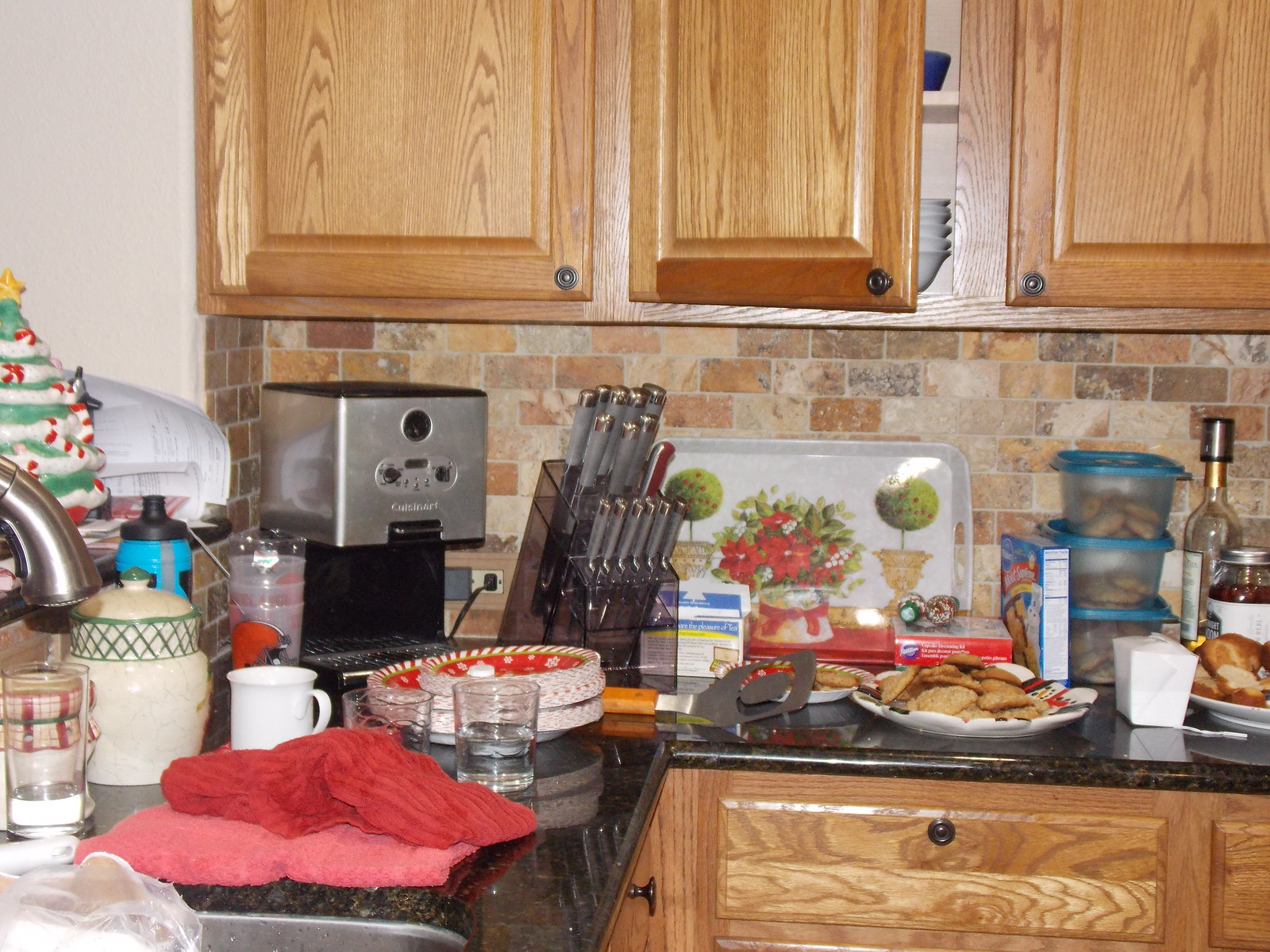The image depicts a bustling kitchen during Christmas time. Dominating the left corner is a charming ceramic Christmas tree, adorned with green and white stripes, red and white ceramic candy canes, and crowned with a gold star. Nearby stands a coffee maker, nestled among an assortment of knives and an array of other items that collectively create a cluttered countertop. The workspace features sleek black granite surfaces and warm wood cabinets, with the middle upper cabinet door left ajar, revealing neatly stacked white bowls inside.

Scattered across the black granite countertop are festive red paper plates and napkins, alongside a tray that holds even more holiday cheer with green topiaries, possibly featuring a poinsettia design in the center. A collection of cookies is artfully displayed on various plates and stored in plastic containers, accompanied by a boxed cake mix and an incongruous Chinese food container.

In addition to these festive treats, a bottle of wine can be spotted towards the right of the scene, suggesting ongoing holiday preparations or celebrations. On the far left side, a sink comes into view, emphasizing the limited corner snapshot of this lively, seasonally-decorated kitchen.